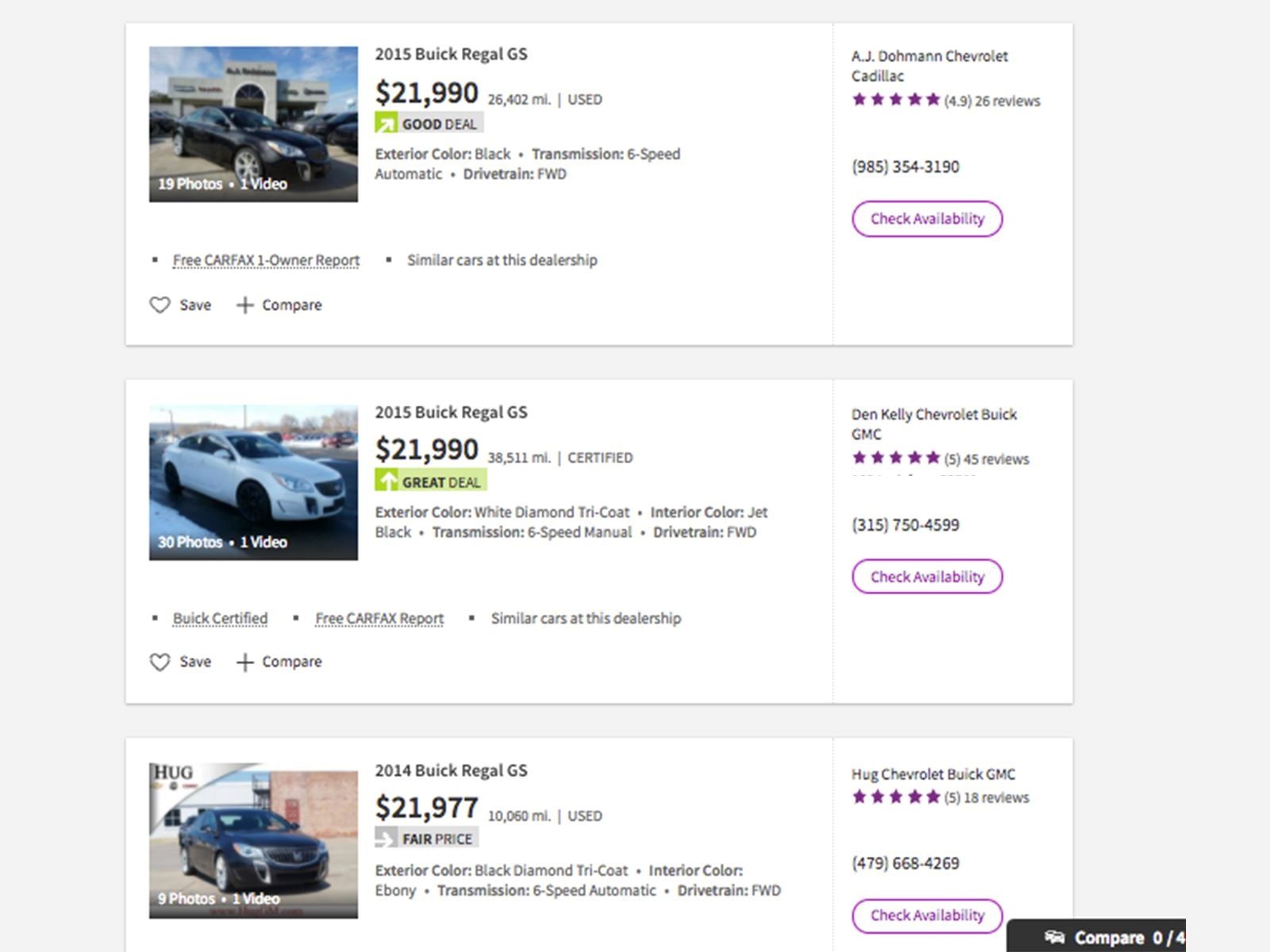A screenshot from a used car dealership website displaying three different cars for sale is shown. 

1. The first car is a **2015 Buick Regal GS** priced at **$21,990**. It has **26,402 miles** on it and is depicted as a good deal. The car is black with a six-speed automatic transmission and a front-wheel drive train. It includes a free CarMax one-owner report. You can save or compare this vehicle, which is available at **AG Dome Chevrolet Cadillac**. The dealership is highly rated with **4.9 stars**. Contact at **985-354-3190** for availability.

2. The second vehicle is another **2015 Buick Regal GS**, also priced at **$21,990** but with **38,511 miles**. This car is certified and marked as a great deal. It has a white exterior with a diamond tri-coat and a jet-black interior. The car features a six-speed manual transmission and front-wheel drive. Additionally, it comes with a free CarMax report. This car can be found at **Don Kelly Chevrolet Buick GMC**, which boasts **45 reviews and five stars**. For more details, call **315-750-4599**.

3. The third car is a **2014 Buick Regal GS** with a price tag of **$21,977** and just **10,000 miles** on it. This used vehicle has a black diamond tri-coat exterior and an ebony interior. It is equipped with a six-speed automatic transmission and front-wheel drive. Available at **Hug Chevrolet Buick GMC**, this dealership has **18 reviews and five stars**. For check availability, contact **479-668-4269**.

Each vehicle listing includes a button to check availability.